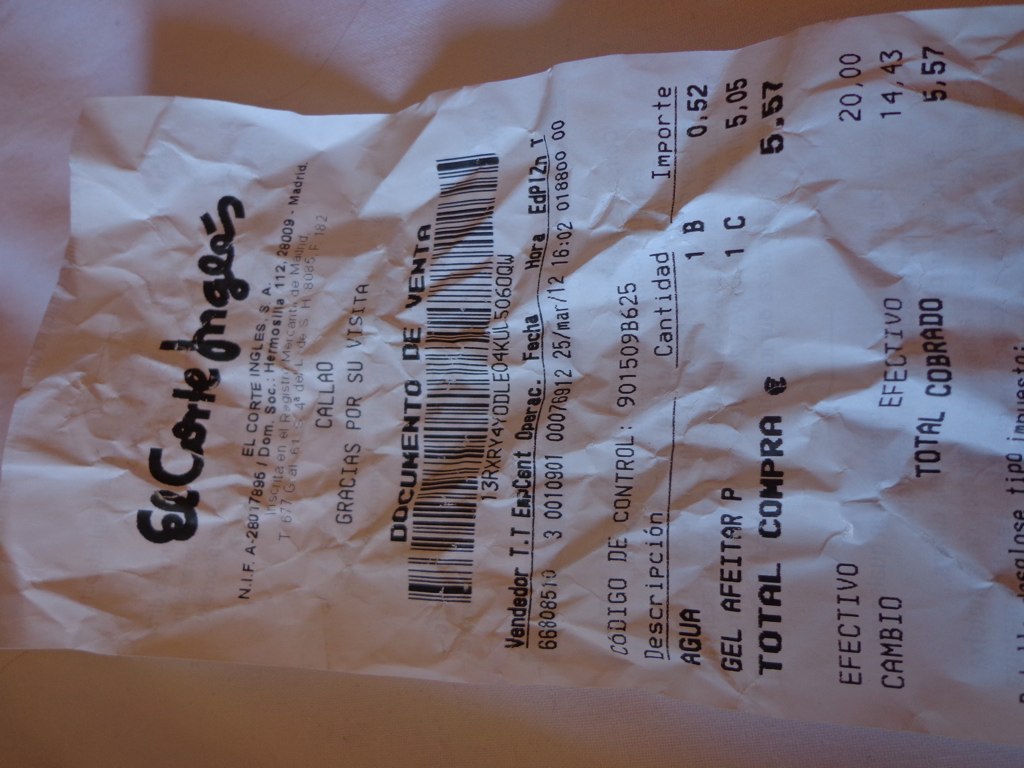This horizontal image showcases a crumpled and subsequently flattened paper receipt from El Corte Inglés, a department store located in Hermosillo, Madrid, Spain. The receipt is positioned sideways, with the bold black lettering at the top, reading "El Corte Inglés," oriented towards the right side of the frame. The receipt, printed with black ink on white paper, rests on a textured, wrinkled pink fabric. The details on the receipt include a message of gratitude, "Gracias por su apoyo," along with a barcode. The transaction recorded indicates a purchase amount of 5.57 euros, paid with a 20-euro note, resulting in 14.43 euros in change.